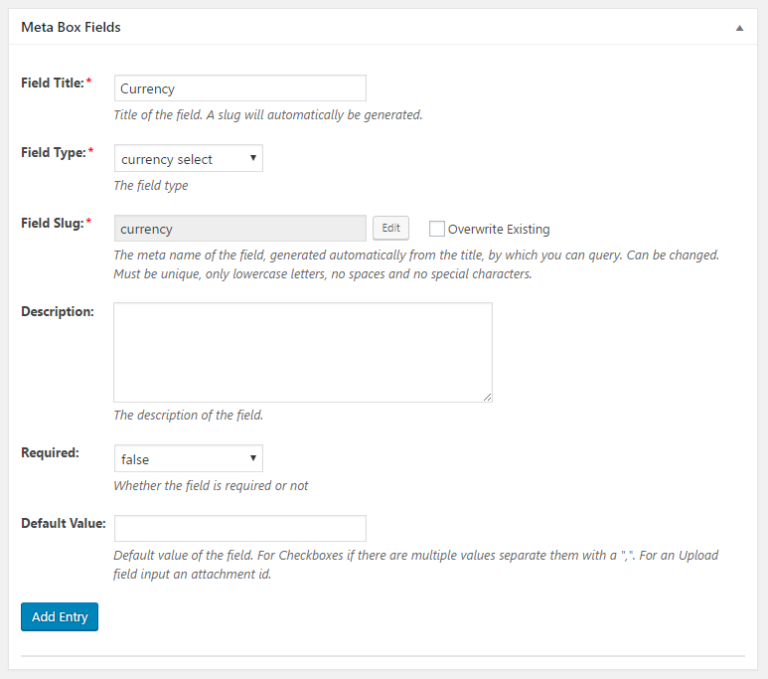The image depicts a detailed Meta Box field form, typically used for social media configurations, presumably powered by Facebook or vice versa. 

- **Top Left Corner**: The title "Meta Box Fields" is prominently displayed.
- **Field Title Section**: Below the title, there's a "Field Title" label, marked with a red asterisk to indicate that it is a mandatory field. The current value specified is "currency." 
  - Adjacent to the field title, there's a description that states "Title of the Field." 
  - A "Slug" for this field is automatically generated.
  
- **Field Type Section**: This section is marked with a red asterisk, denoting that it is mandatory. It features a dropdown menu.
  - Below this, the "Slug" field for "currency" is displayed within a light gray box, accompanied by an "Edit" button to its right.
  - There is also a checkbox option labeled "Overwrite Existing."

- **Description Section**: An input box allows for an optional description (as indicated by the absence of a red asterisk).

- **Required Section**: 
  - A dropdown box labeled "Required" currently shows a value of "false," allowing the user to specify whether the field is required or not.

- **Default Value Section**: 
  - Here, there is an input field labeled "Default Value" which is currently blank. 
  - It notes that for a checkbox with multiple values, values should be separated by quotations. For an upload field, input should be an attachment ID.

- **Bottom Section**: 
  - At the bottom left, a blue "Add Entry" button is available, inviting the user to submit the form.